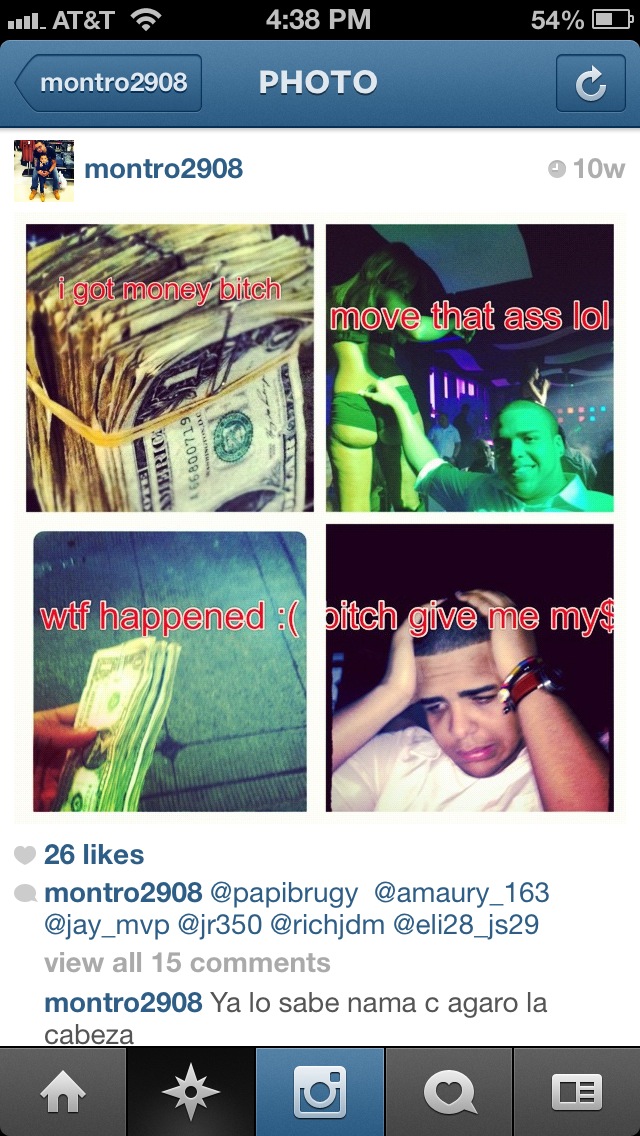This image appears to be a screenshot from an Instagram post made by the user Montro2908. His profile features an avatar of a Hispanic man crouched down, holding his son. The overlay indicates an AT&T connection with 54% battery at 4:30 PM. The post is a meme composed of four distinct images: 

1. The top-left shows a thick wad of ragged dollar bills bound by a rubber band with the text "I got money, bitch."
2. The top-right features a Hispanic man in a strip club, seen placing a dollar bill into a stripper’s panties. Another stripper is visible in the darker background, accompanied by the text "move that ass, LOL."
3. The bottom-left shows a significantly thinner stack of dollar bills, about a third the size of the first stack, with the caption "WTF happened," followed by a frown emoji.
4. The bottom-right portrays the same Hispanic man looking sad and holding his head, wearing a wristband, with the text "bitch, give me my money."

The post has garnered 26 likes and 15 comments, all appearing to be in Spanish. Standard Instagram interface elements such as the refresh icon and sharing options are also visible.